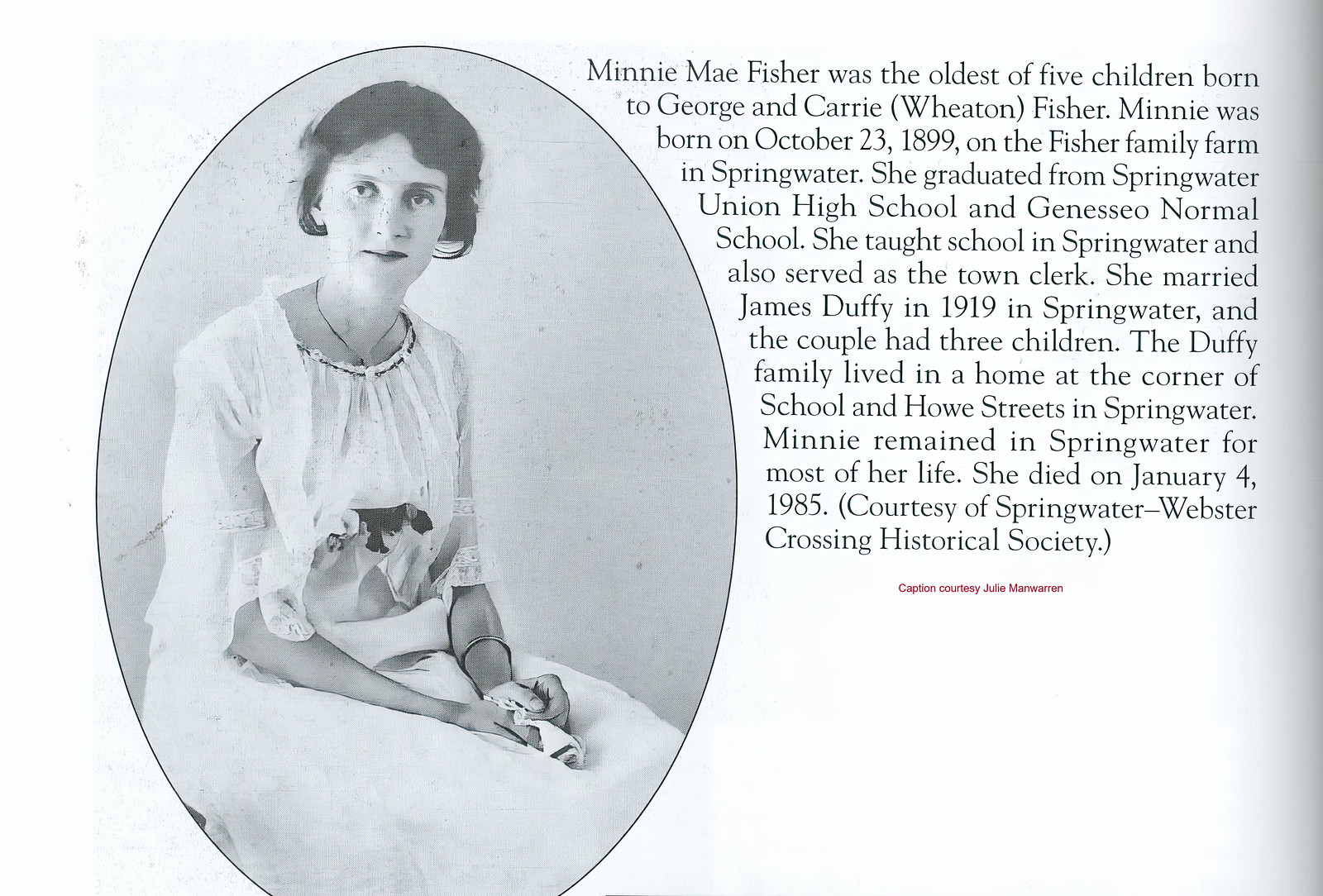This black-and-white photograph, framed in an oval, depicts Minnie Mae Fisher, born on October 23, 1899, the eldest of five children of George and Carrie Wheaton Fisher. The young woman, with short brunette hair, is captured in a formal white satin gown, adorned with a necklace and a bracelet on her left arm. Minnie is seated with her hands resting in her lap, delicately holding what appears to be a cloth or rolled-up hat. Her gaze is slightly away, yet towards the camera. The image, taken from a book on white paper, is accompanied by text detailing Minnie’s life: she grew up on the Fisher family farm in Springwater, graduated from Springwater Union High School, and Geneseo Normal School, taught school in her hometown, and served as the town clerk. In 1919, she married James Duffy, with whom she had three children. The Duffy family resided at the corner of School and Howie Streets in Springwater, where Minnie remained for most of her life, until her passing on January 4, 1985. This caption also mentions that the image and text are courtesy of the Springwater-Webster Crossing Historical Society, and includes an additional note in red ink: "Caption courtesy Julie Marwarn."